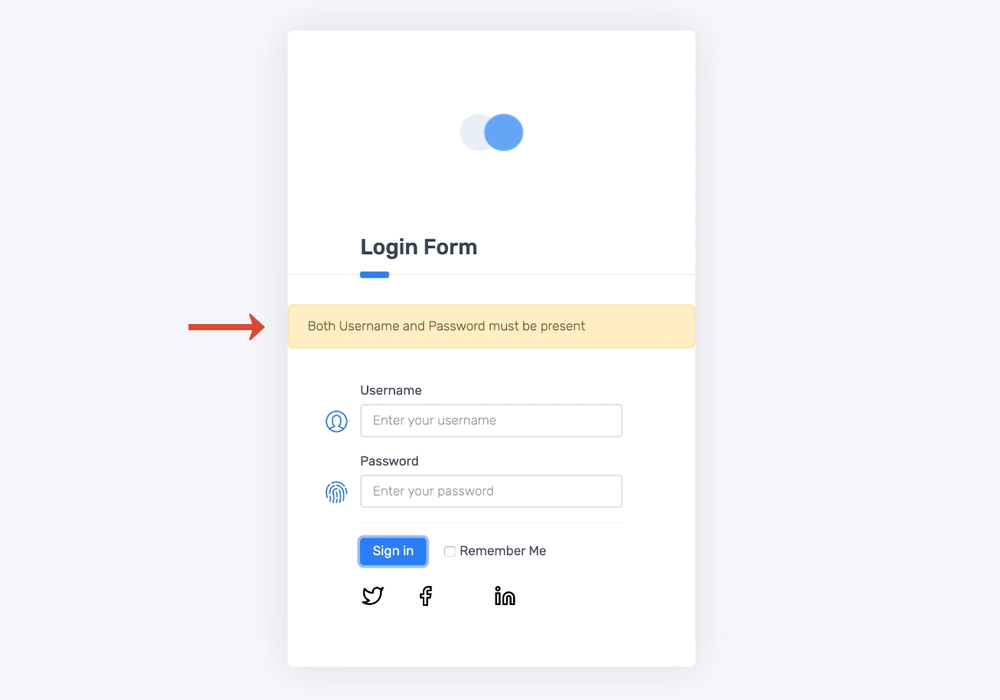The image appears to be a screenshot of a login interface on a cell phone screen. Dominating the visual is a light gray rectangle that spans horizontally across the image. At the center of this gray rectangle lies a vertically oriented white rectangle. 

At the top of this white rectangle, there's a blue circle resembling the typical on-off switch that turns blue upon activation. Just below this circle, the text "Login Form" is prominently displayed, with a subtle blue underline beneath the word "Login". 

Immediately following this, there's a yellow box containing the alert text "Both username and password must be present". A red arrow points towards this line from the left, drawing attention to the message.

Further below in the white rectangle, the text "Username" is labeled above a text box prompting the user to "Enter Your Username". Similarly, "Password" appears above another text box that says "Enter Your Password".

Under these fields, there is a blue rectangle featuring "Sign In" as the clickable button. Adjacent to it lies a small blank square accompanied by the label "Remember Me".

At the bottom of the white section, various social media icons are displayed: a bird symbol for Twitter, an "F" for Facebook, and an "IN" symbol likely representing LinkedIn.